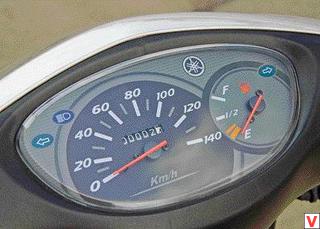This image captures the dashboard of a vehicle, possibly a car or a boat, featuring an analog speedometer as the central instrument. The speedometer display ranges from 0 to 140 kilometers per hour, clearly marked with numerical increments. To the right of the speedometer, partially embedded within it, is a smaller, round fuel gauge that measures fuel levels from empty to full. Notably, the fuel gauge needle is currently indicating below empty, suggesting it might be powered off or the tank is genuinely low.

In addition to these primary gauges, there are several indicator lights present. On the left side, a left turn signal light is visible, mirrored by a right turn signal light on the right side. Other indicators include a headlamp icon and a symbol with crisscrossed white bars located between the speedometer and the fuel gauge, though its exact purpose is unclear. The entire ensemble of gauges and indicators are designed in a distinctive, eye-catching manner; the shape of the gauge cluster collectively mimics the form of a large eyeball. This unique design adds an element of visual interest to the dashboard's functional layout.